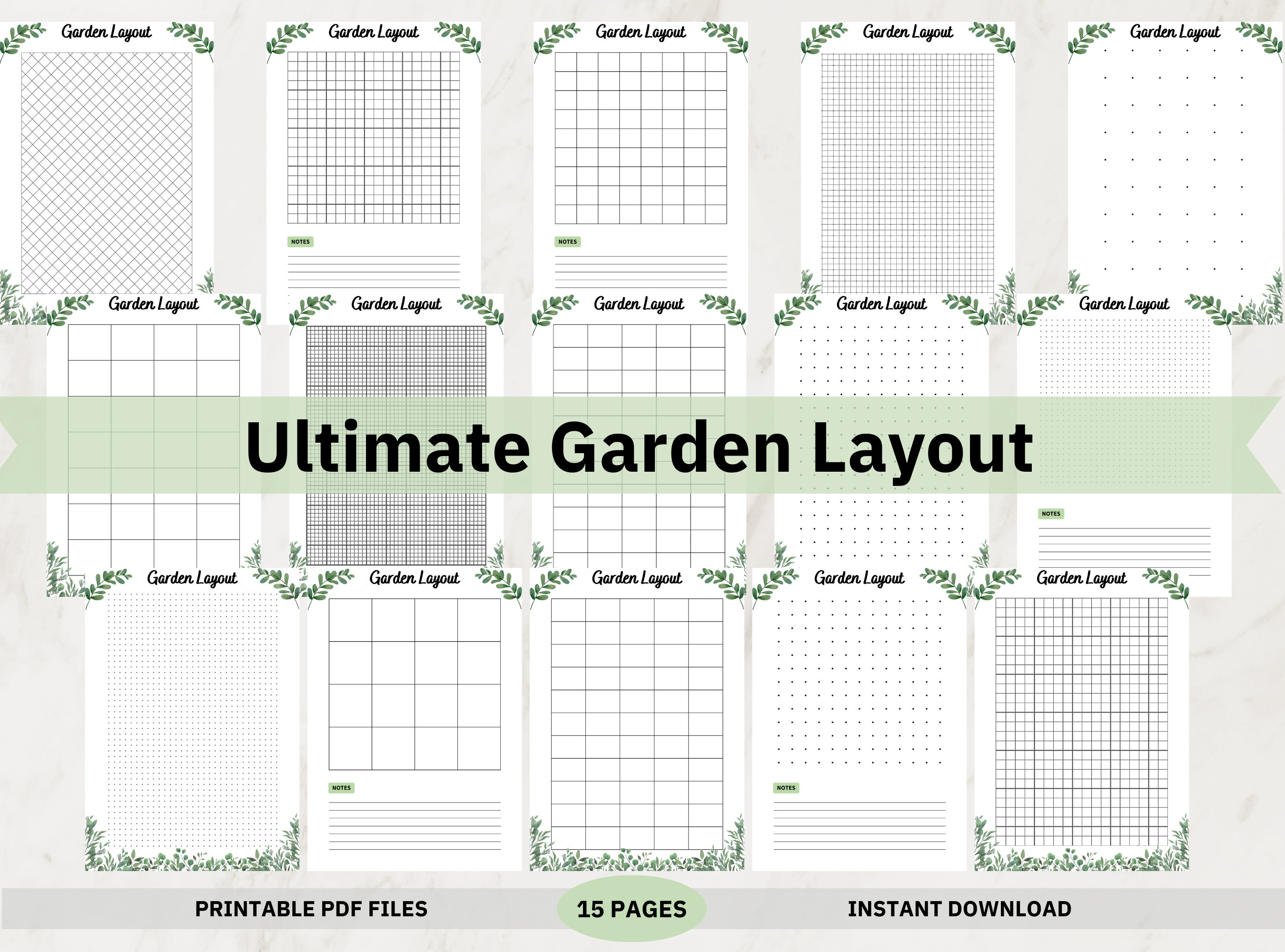This promotional image displays a 15-page set of printable PDF templates titled "The Ultimate Garden Layout." Each page features a detailed grid for planning garden plots, with leafy designs adorning the borders to complement the gardening theme. The templates are arrayed in a neat matrix of five columns by three rows. A green horizontal banner across the center of the image prominently displays the title "The Ultimate Garden Layout" in black text. At the bottom, a gray bar on the left indicates "Printable PDF files," while a green oval in the center mentions "15 pages," and the text "Instant download" appears on the right. Each template page is depicted against a cream-gray background, showcasing varied grid designs to help users organize their spring or summer garden layouts effectively.